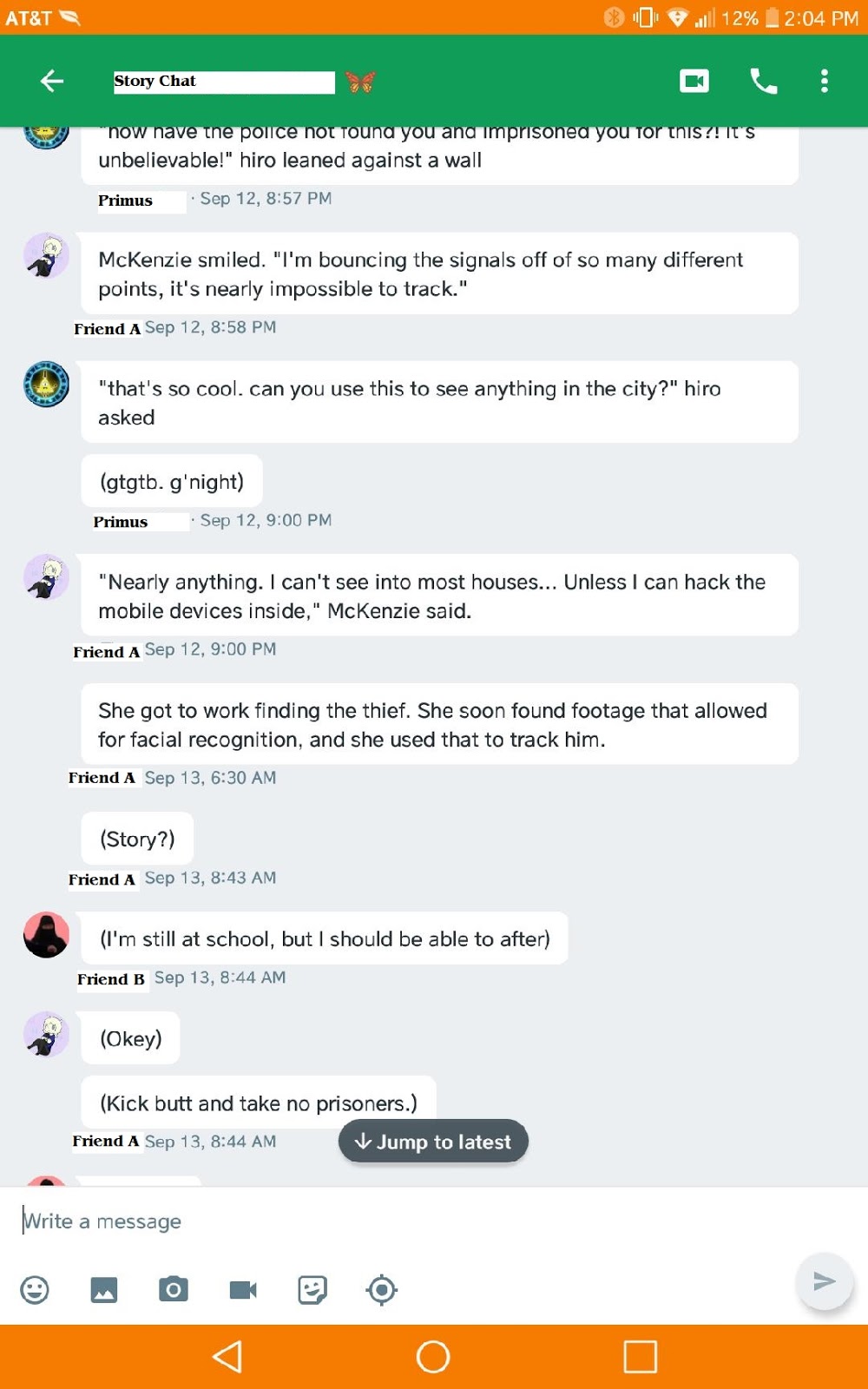The image captured from a cell phone screen during a story chat session features a visually structured user interface with distinct details. At the very top of the screen, an orange rectangular status bar displays standard cell phone indicators. It shows that the network provider is AT&T, and also includes icons for a leaf, Bluetooth, vibration, Wi-Fi, signal bars, and a battery indicator with 12% remaining, displayed as a partially filled orange battery icon. Additionally, the time displayed is 2:04 PM.

Beneath the status bar, a green rectangular header labeled "Story Chat" is present, adorned with a butterfly icon at its edge. This section transitions into a conversation area where the chat narrative begins. The dialogue opens with a question about law enforcement: "How have the police not found you and imprisoned you for this? It's unbelievable." The scene depicts Hero leaning against a wall, followed by Mackenzie's reply: "Mackenzie smiled. I'm bouncing the signals off of so many different points it's nearly impossible to track." A subsequent query from Hero reads: "That's so cool, can you use this to see anything in the city?" Further down, a brief message "GTGTB. Gnight" appears in the chat. The dialogue continues with Mackenzie explaining her technological prowess: "Nearly anything. I can't see into most houses unless I hack the mobile devices inside," and it details her effort to locate the thief. She successfully identifies the culprit through facial recognition from collected footage, using this advanced tracking to follow his movements.

Finally, the screen's design concludes with a red-orange rectangular area at the very bottom, marking the end of the visible chat session.